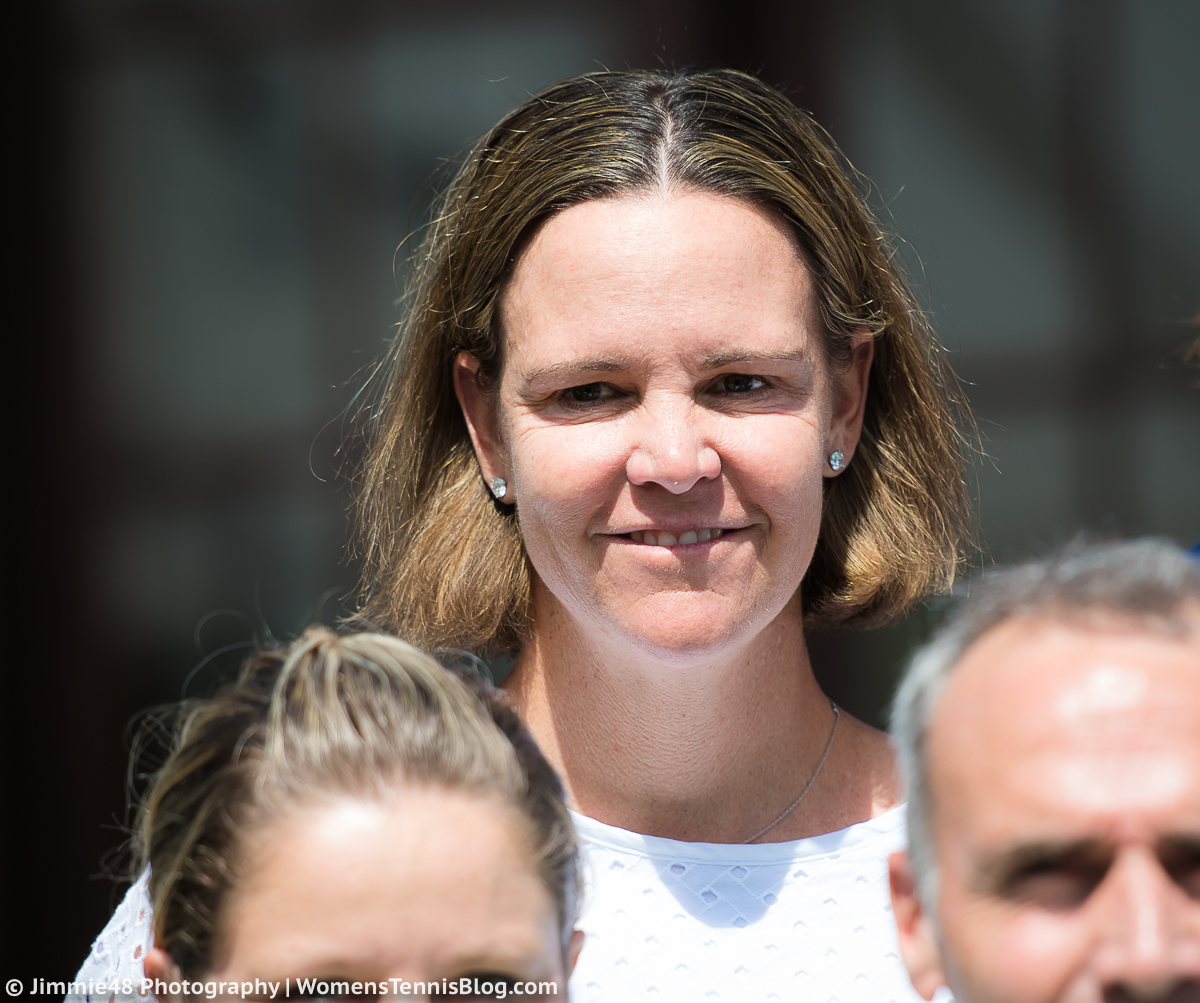In this image, the background is mostly blurred, making it difficult to discern any specific details or setting, though it appears to be taken outdoors in the middle of the day. The primary focus is on three people. At the bottom of the image, partially cut off, is a man with gray hair, revealing about 60% of his face, and a woman with blonde and brown hair, visible only from her eyes up. Dominating the center is a woman with light brownish-blonde hair pushed back behind her ears. She is smiling directly at the camera, wearing diamond earrings, a necklace, and a white checkered shirt. The bottom left of the image has the text "Jimmy48 Photography, womens tennis blog dot com." The visible colors in the image are various shades of black, green, brown, tan, white, and gray.